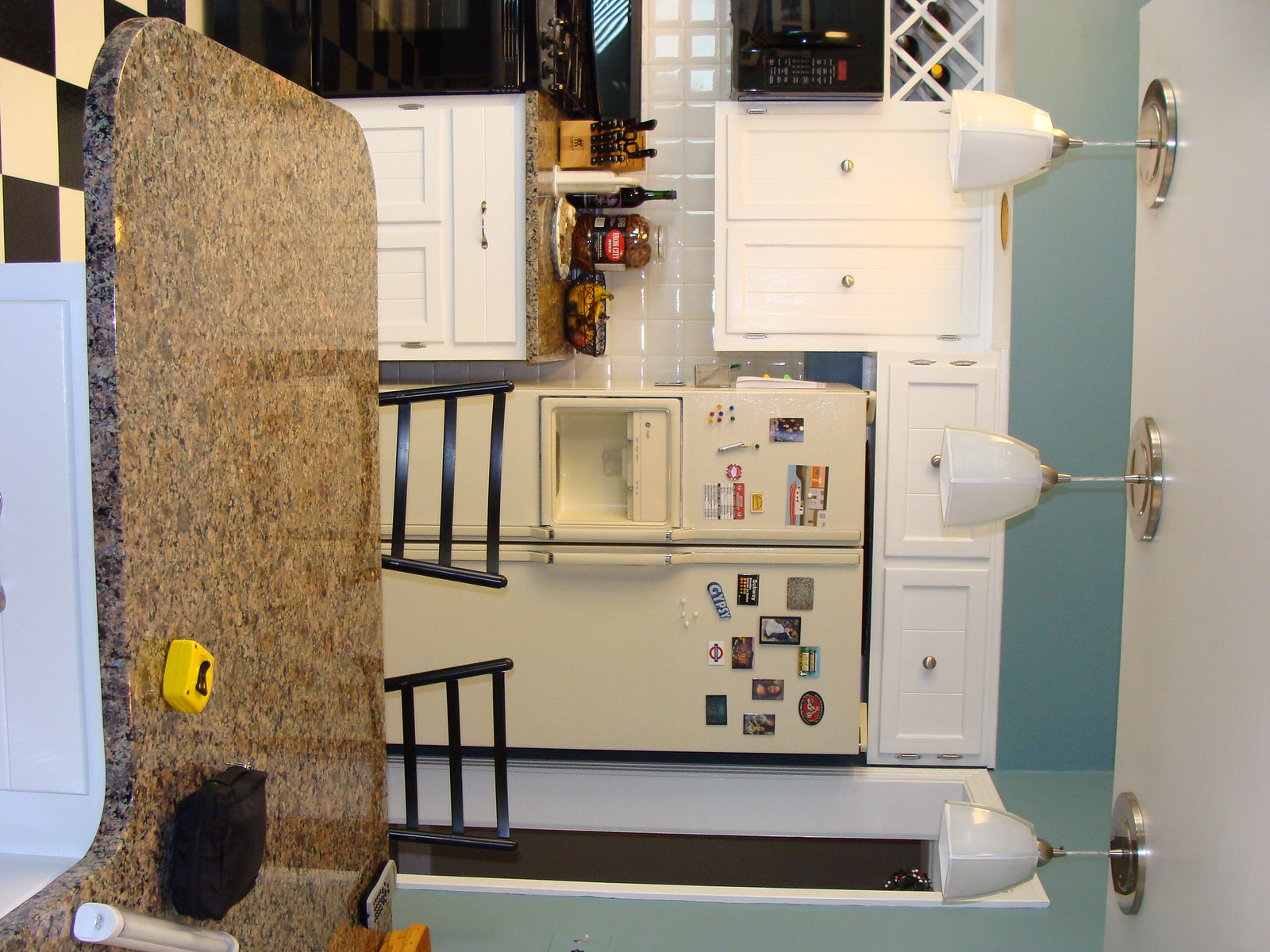This photograph captures the interior of a kitchen, though the image is rotated such that the ceiling appears on the right side. Dominating the scene are sleek, white, square-shaped pendant lights hanging above a curved granite countertop, which features a rich brown hue accented with black speckles. The countertop, suggestive of a bar area, is flanked by at least two chairs with horizontal wooden backs.

Minimal clutter is present on the countertop, with a yellow tape measure and a black object clearly visible. The kitchen floor is adorned with striking black and white checkered tiles. Behind the bar area, white wooden cabinets with vertical patterns and silver knobs are neatly arranged, providing a backdrop. A side-by-side refrigerator, creamy in color and equipped with an ice dispenser, is adorned with an assortment of magnets, adding a personalized touch to the scene.